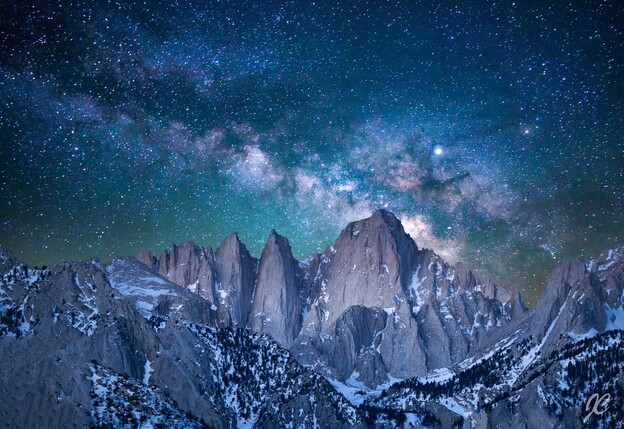The image is a highly detailed, digital painting of a rocky mountain range with some snowy peaks interspersed. The jagged, steep mountains extend upwards into a striking, starry night sky. Pine trees are scattered across the mountainsides, adding natural texture. The nighttime setting is accentuated by a breathtaking cosmic display in the background, featuring the Milky Way with an ethereal mix of blue, green, and even some brown hues, creating a space dust effect. Despite some clouds, the sky remains densely populated with stars, and a prominent, bright star adds a focal point. The overall color palette leans heavily toward blue and gray tones, enhancing the serene yet majestic atmosphere. Additionally, a logo reading "JC" is subtly placed in the lower right corner of the image, suggesting the artist's credit.